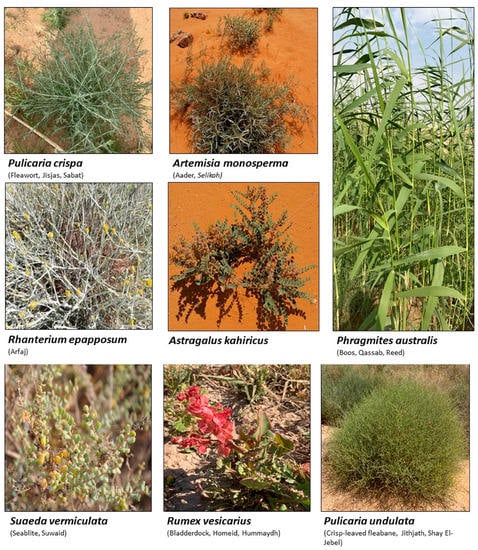This is a detailed diagram showcasing eight different desert plants, each meticulously labeled with both their common and scientific names. The top left plant is Pulicaria crispa, commonly known as fleawort. To its right is Artemisia monosperma, followed by Astragalus cahiricus below it. Positioned left of Astragalus cahiricus is Ranterium epapposum, known as arfage. Phragmites australis, also called reed, is to the far right. Below it is Pulicaria undulata, identified as crisp leaf fleabane. Rumex vesicarius, or bladder dock, is to the left of Pulicaria undulata. Finally, on the bottom left is Suaeda vermiculata, known as sea blight. The ground behind each plant is dry sand, highlighting their adaptation to arid environments. Notably, some plants exhibit sparse flowers: the middle left features a few yellow flowers, the middle bottom has some red flowers, and the bottom left showcases small yellow balls.